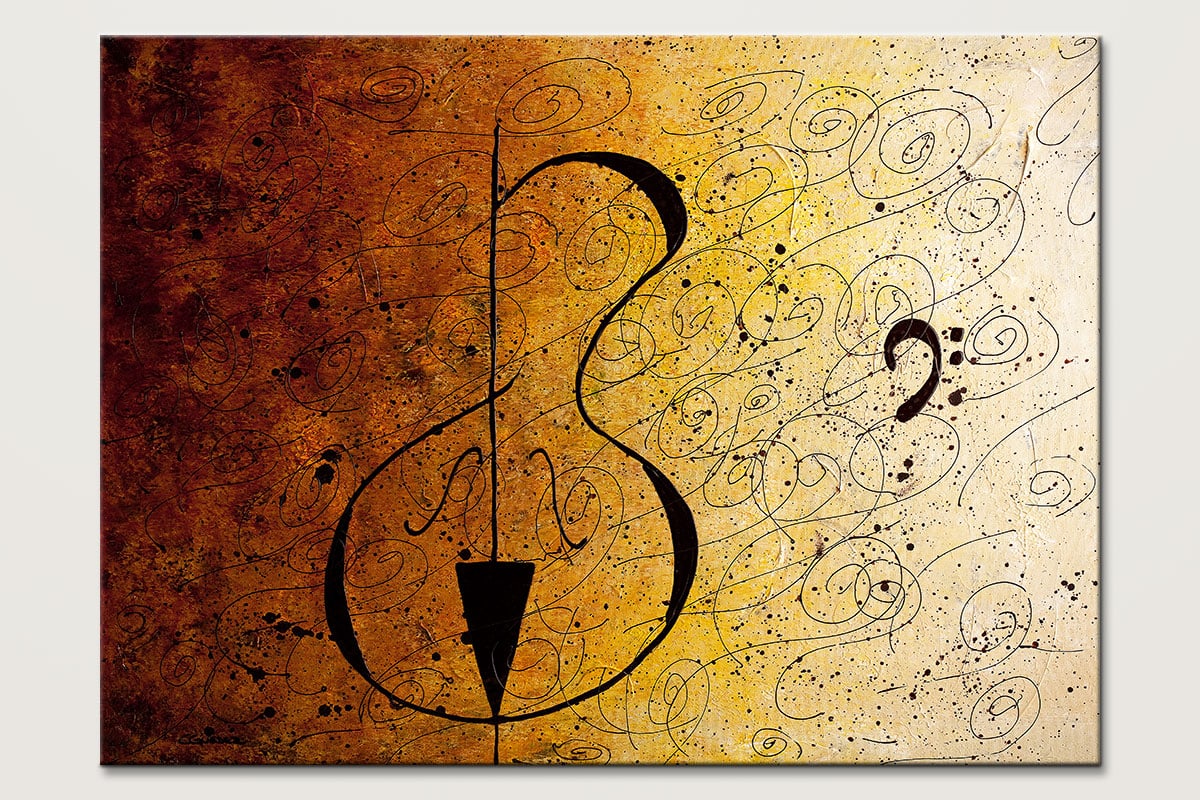The image appears to be a photograph of an abstract painting, characterized by a musical theme. Dominating the center of the composition is a prominent black symbol, reminiscent of a musical note or time signature, boldly standing out against the background. Throughout the painting, similar black squiggles and lines are visible, becoming more evident as they extend towards the right side. The background exhibits a gradient, transitioning from a dark, dirty brown on the far left, through shades of metal, clay, orange, and yellow, until it becomes a pale, creamy white on the far right. This color shift enhances the sepia-toned aesthetic of the painting. The intricate patterns and the prominent central symbol collectively suggest an abstract representation of musical elements.